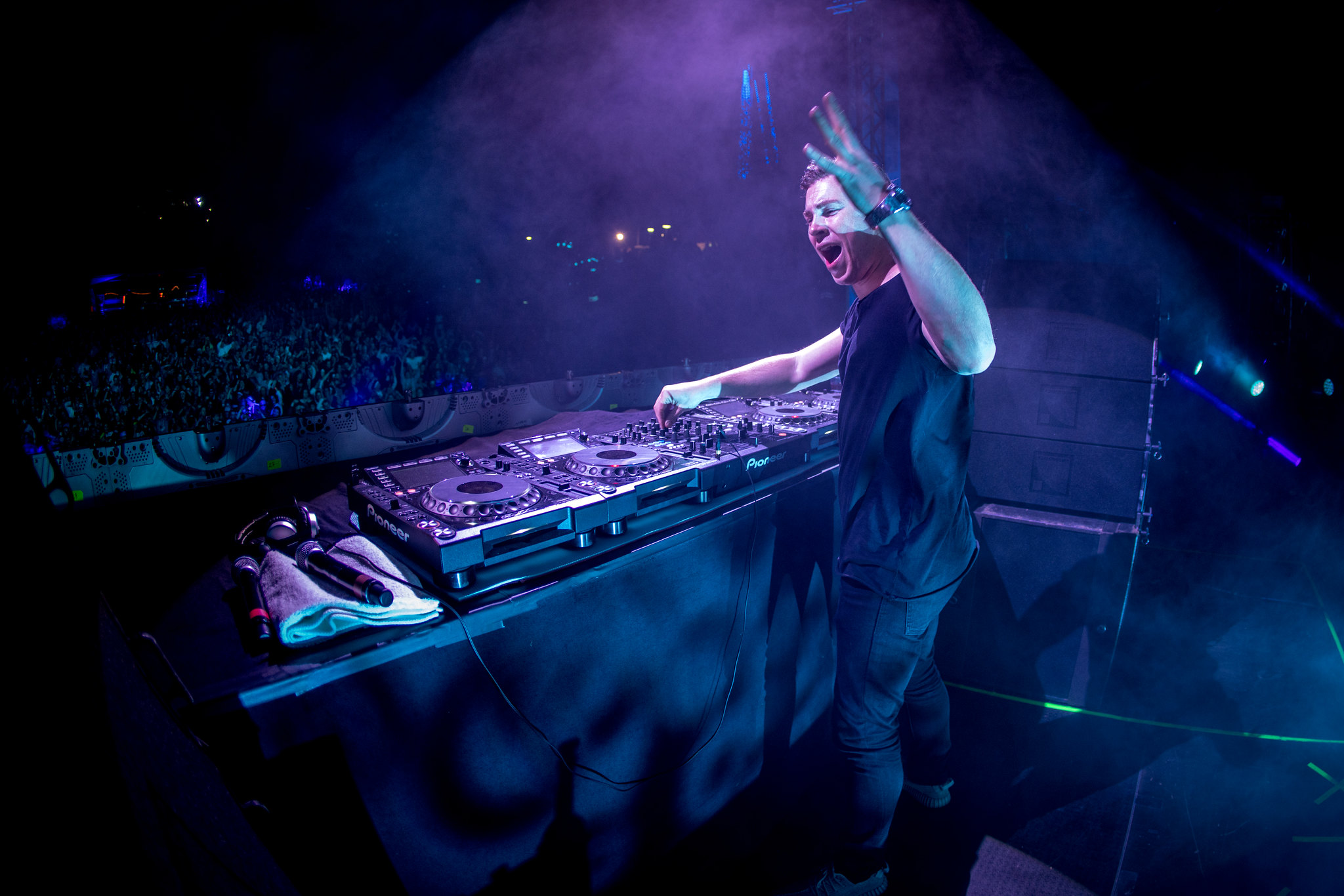In this dynamic concert photo, DJ Hardwell, a young white male, commands the stage, dressed in black jeans and a black t-shirt. Taken from behind and slightly to the side, the shot captures him intensely engaged with his DJ mixing table. His right hand expertly maneuvers the knobs on the extensive DJ equipment before him, which includes several turntables and an assortment of audio gear. On the left side of the table, a microphone and a pair of headphones rest atop a towel. His left arm is raised high, and a black watch adorns his wrist, while his mouth is wide open, either shouting to the crowd or singing along with the music. The dark, smoky atmosphere is pierced by vibrant blue and white lights, heightening the sense of an energetic live performance. Below the stage, a distant audience is bathed in the ambient glow, eagerly absorbing the electrifying show.